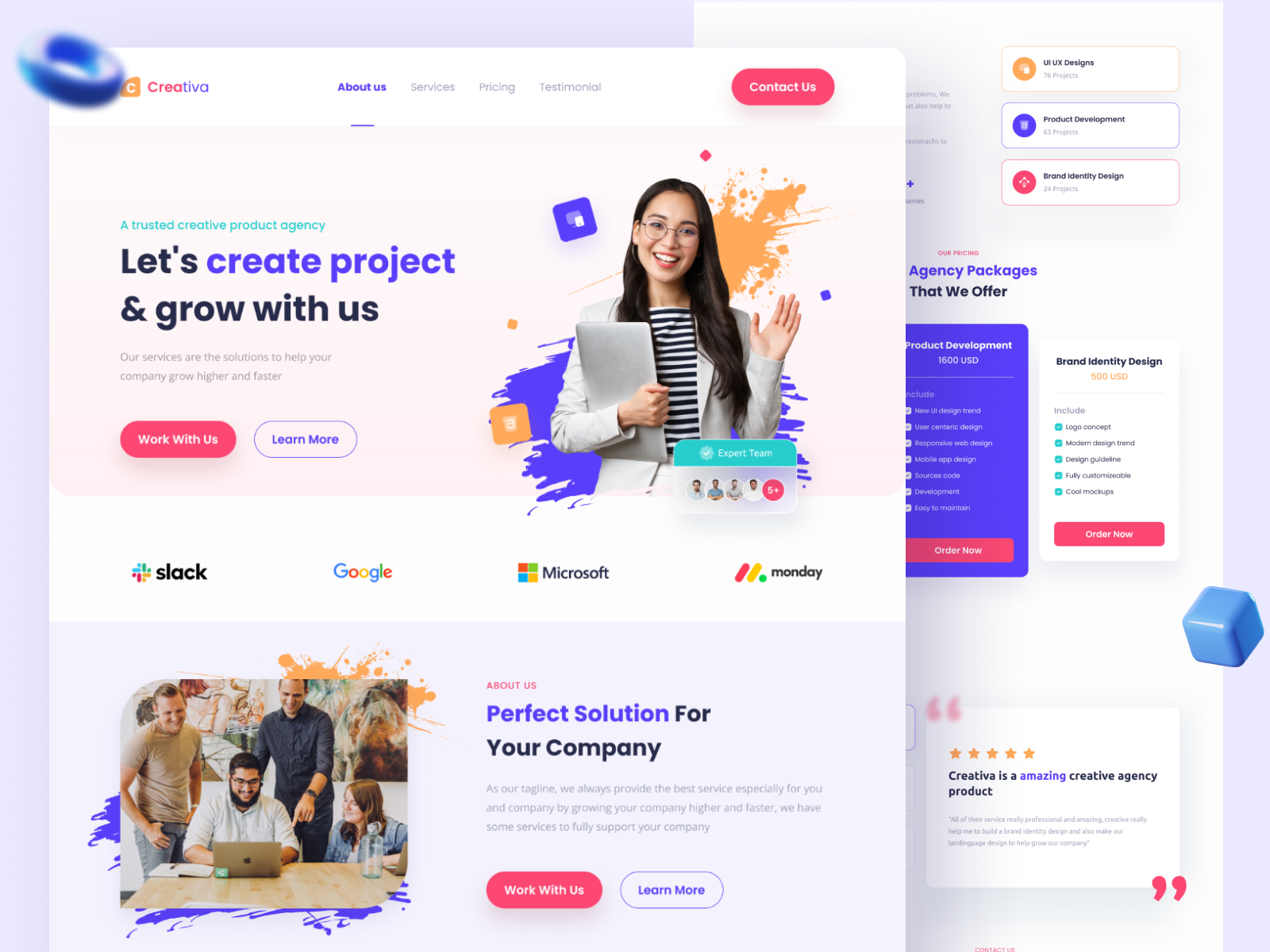This image is a detailed screenshot from a web page of Creativa, a creative product agency. In the top left-hand corner, the word "Creativa" is displayed prominently, followed by navigation options for "About Us," "Services," "Pricing," and "Testimonial." Next to these options is a red oval button labeled "Contact Us" in white text.

Below the navigation, there is a photograph featuring a young woman with glasses and long dark hair. She is dressed in a striped shirt and a gray blazer and is holding a large tablet computer in her arm while extending her other hand as if to wave hello. The backdrop of the photograph features vibrant splashes of orange and purple paint.

To the left of the photograph, in teal-colored text, it reads "A Trusted Creative Product Agency," followed by a call-to-action message, "Let's Create Projects and Grow With Us. Our services are the solutions to help your company grow higher and faster." Below this message are two buttons: a red oval labeled "Work With Us" and a purple oval labeled "Learn More."

Further down, a row of logos for prominent companies like Slack, Google, Microsoft, and Monday is displayed. Underneath the logos, the text reads "About Us: Perfect Solution for Your Company. Work With Us or Learn More."

On the far right side of the screenshot, part of another section is visible, which lists services such as "UI/UX Designs," "Product Development," "Brand Identity Design," and "Agency Packages That We Offer." Pricing details include "Product Development for $1,600 USD, Order Now" and "Brand Identity Design for $500 USD, Order Now." A testimonial quote at the bottom praises the agency, stating, "Creativa is an amazing creative agency product."